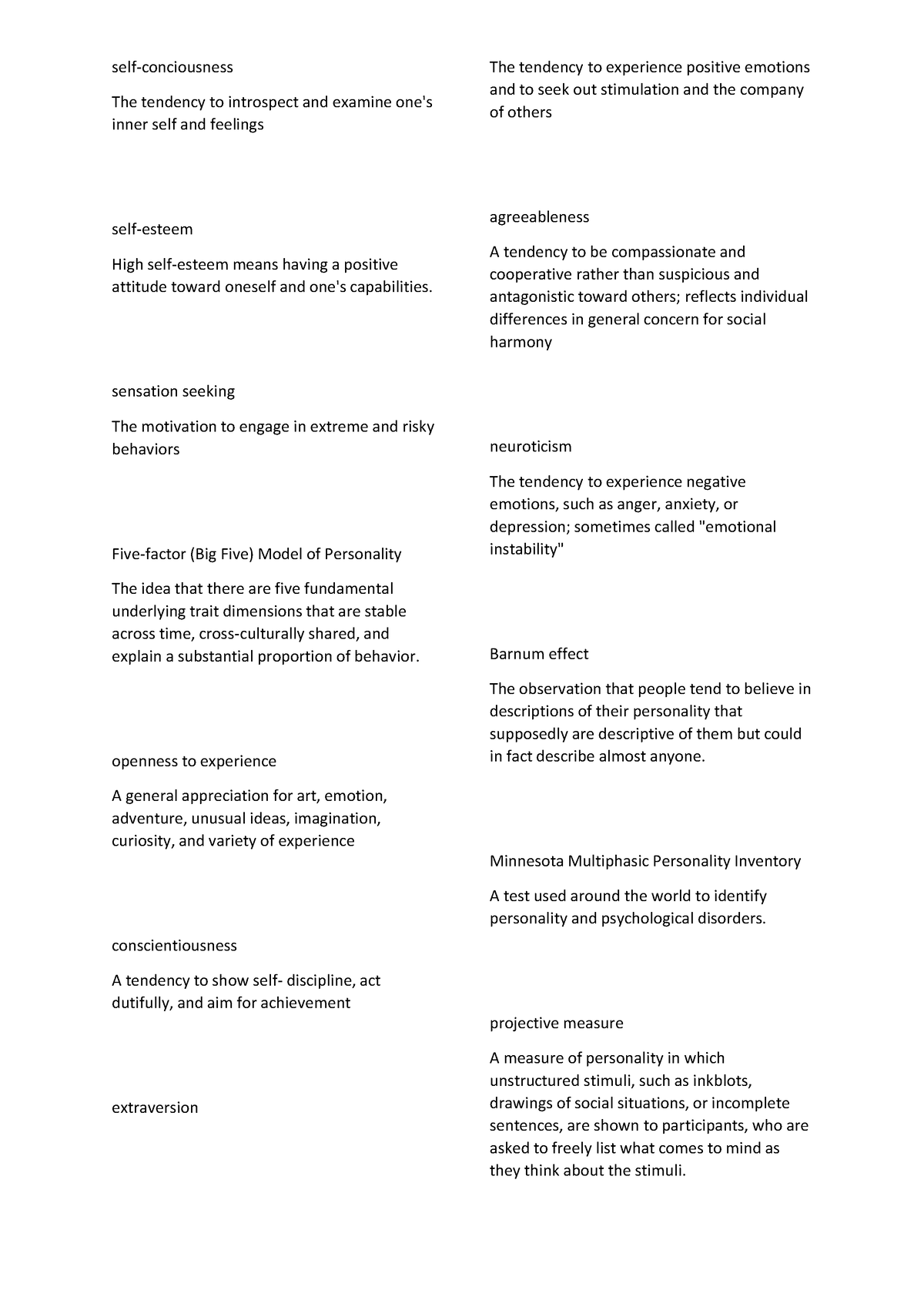This is a detailed screenshot of a self-help text, divided into two vertical columns of text. 

The left column discusses the following personality traits and models:
1. **Self-Consciousness**: The tendency to introspect and examine one's inner self and feelings.
2. **Self-Esteem**: High self-esteem involves having a positive attitude towards oneself and one's abilities.
3. **Sensation-Seeking**: The motivation to engage in extreme and risky behaviors.
4. **Five-Factor (Big Five) Model of Personality**: The concept that there are five fundamental underlying trait dimensions that are stable over time, shared across cultures, and explain a significant proportion of behavior.
   - **Openness to Experience**: A general appreciation for art, emotion, adventure, unusual ideas, imagination, curiosity, and variety of experience.
   - **Conscientiousness**: A tendency to show self-discipline, act dutifully, and aim for achievement.
   - **Extroversion**: The text cuts off here.

The right column continues with the description of personality traits and measures:
5. **Extroversion (continued)**: The tendency to experience positive emotions and to seek out stimulation and the company of others.
6. **Agreeableness**: The tendency to be compassionate and cooperative rather than suspicious and antagonistic towards others, reflecting individual differences in general concern for social harmony.
7. **Neuroticism**: The tendency to experience negative emotions such as anger, anxiety, or depression, sometimes referred to as emotional instability.
8. **Barnum Effect**: The observation that people tend to believe descriptions of their personality that appear to be personalized but could, in fact, apply to almost anyone.
9. **Minnesota Multiphasic Personality Inventory (MMPI)**: A widely used test to identify personality and psychological disorders.
10. **Projective Measure**: A method of assessing personality where unstructured stimuli such as inkblots, drawings of social situations, or incomplete sentences are shown to participants, who are then asked to freely list what comes to mind as they think about the stimuli.

This detailed explanation encapsulates various aspects of personality traits and assessment tools discussed in the text.